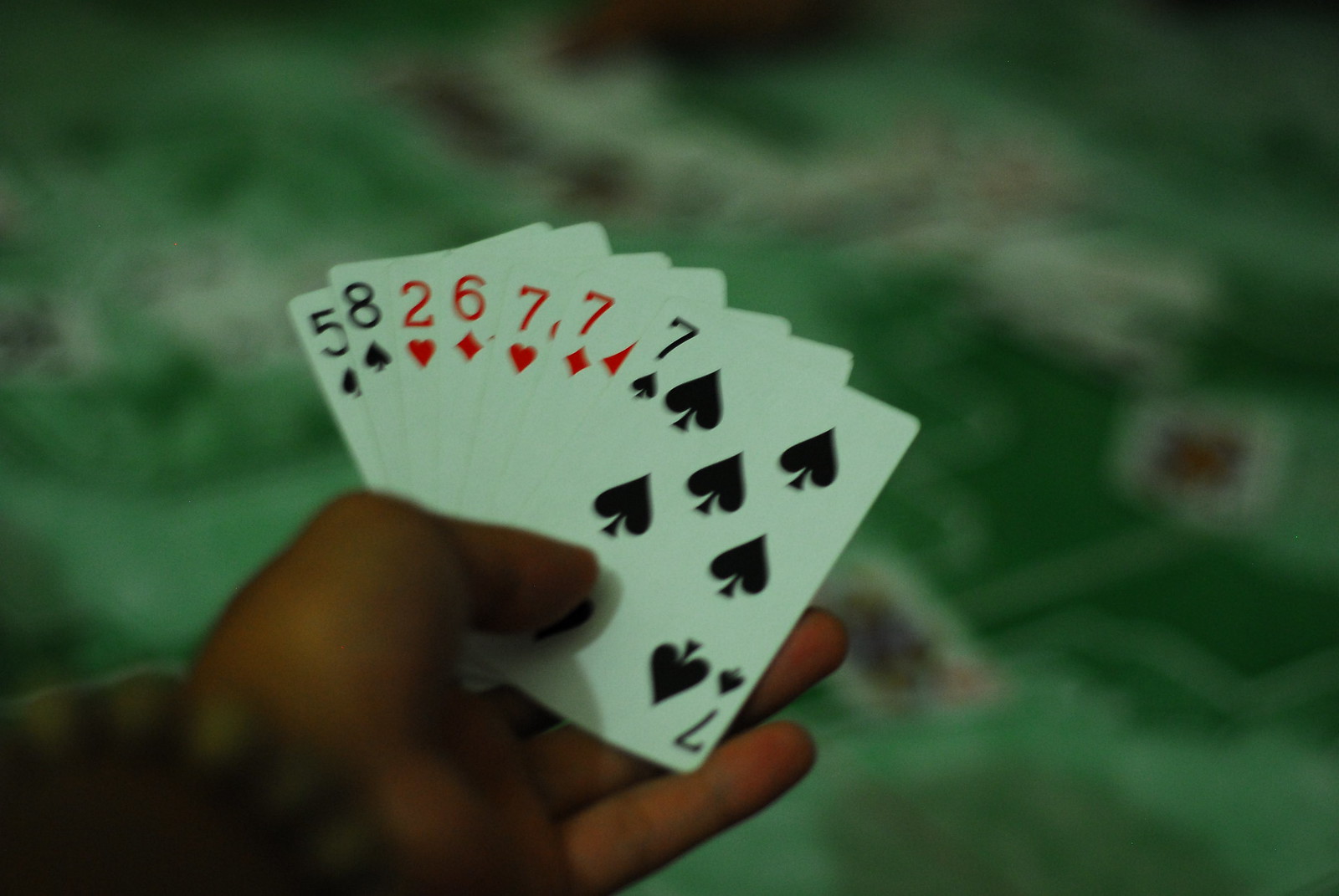A hand adorned with a bracelet of round beads holds a fanned set of seven playing cards over a blurry background of a green felt card table, likely depicting a card game such as Poker or Seven-Card Stud. Alongside the clearly visible seven of spades, six other cards can be identified: the five of spades, eight of spades, two of hearts, six of diamonds, seven of hearts, and seven of diamonds. The cards are fanned in such a way that only their upper left corners are visible, rendering the symbols and suits mostly indistinct except for the well-defined seven of spades on the far right, characterized by its specific spade arrangement. The table shows other indistinct cards and blurry shapes, hinting at possible face cards and another player, yet the overall scene remains unclear.